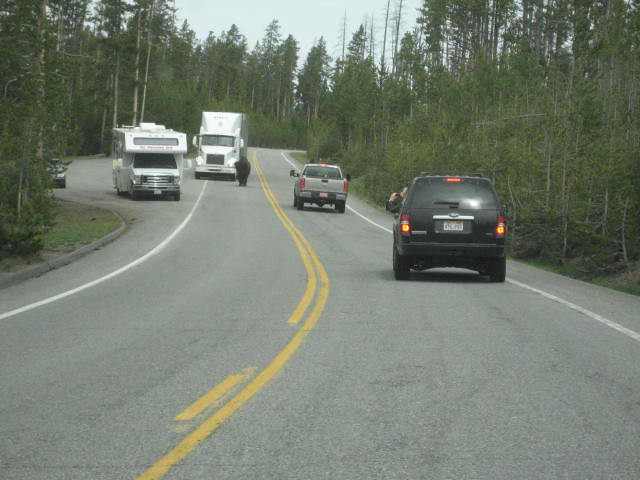This color photograph captures a detailed scene of a winding two-lane road surrounded by tall trees under a partially cloudy, yet bright daytime sky. Positioned slightly uphill and taken from what seems to be a car, though no interior is visible, the image features several vehicles and road elements. On the right-hand lane heading forward, there's a black car followed by a gray 18-wheeler truck. The black car appears to be braking, distinguished by its illuminated brake lights. Meanwhile, in the pullout area on the left side of the road, a white SUV is seen re-entering the roadway. Up ahead in the left lane, a white commercial truck, or 18-wheeler, is advancing, and in front of it, possibly standing on the roadside, is a person dressed in black, seemingly observing traffic. There's also a white camper van in the same pullout area partially obscured by the trees. The road itself, curving to the right before extending uphill, is gray with distinct yellow middle lines and white lines marking the lanes and pullout areas. The image, though slightly blurry and underexposed, vividly showcases the serene yet dynamic roadside scene.